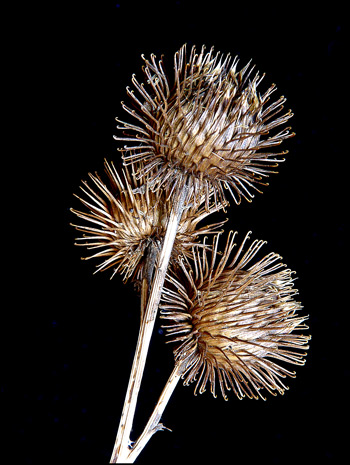This is a close-up photograph capturing three dried thistles set against a pitch-black background. The central thistle stands the tallest, flanked by two shorter ones, with the rightmost thistle slightly tilting to the right and the leftmost one leaning away from the viewer. Each thistle, attached to a faint light brown stem, ends in a spherical bulb covered in numerous tiny, slightly curved barbs, resembling prickly hedgehogs. The brown bulbs are textured and intricate, with barbs sticking out at angles, illuminated by a touch of studio light that accentuates their details. This stark, detailed depiction highlights the distinctive, spiky nature of the thistles, reminiscent of the sticky burrs one might encounter walking through the woods.